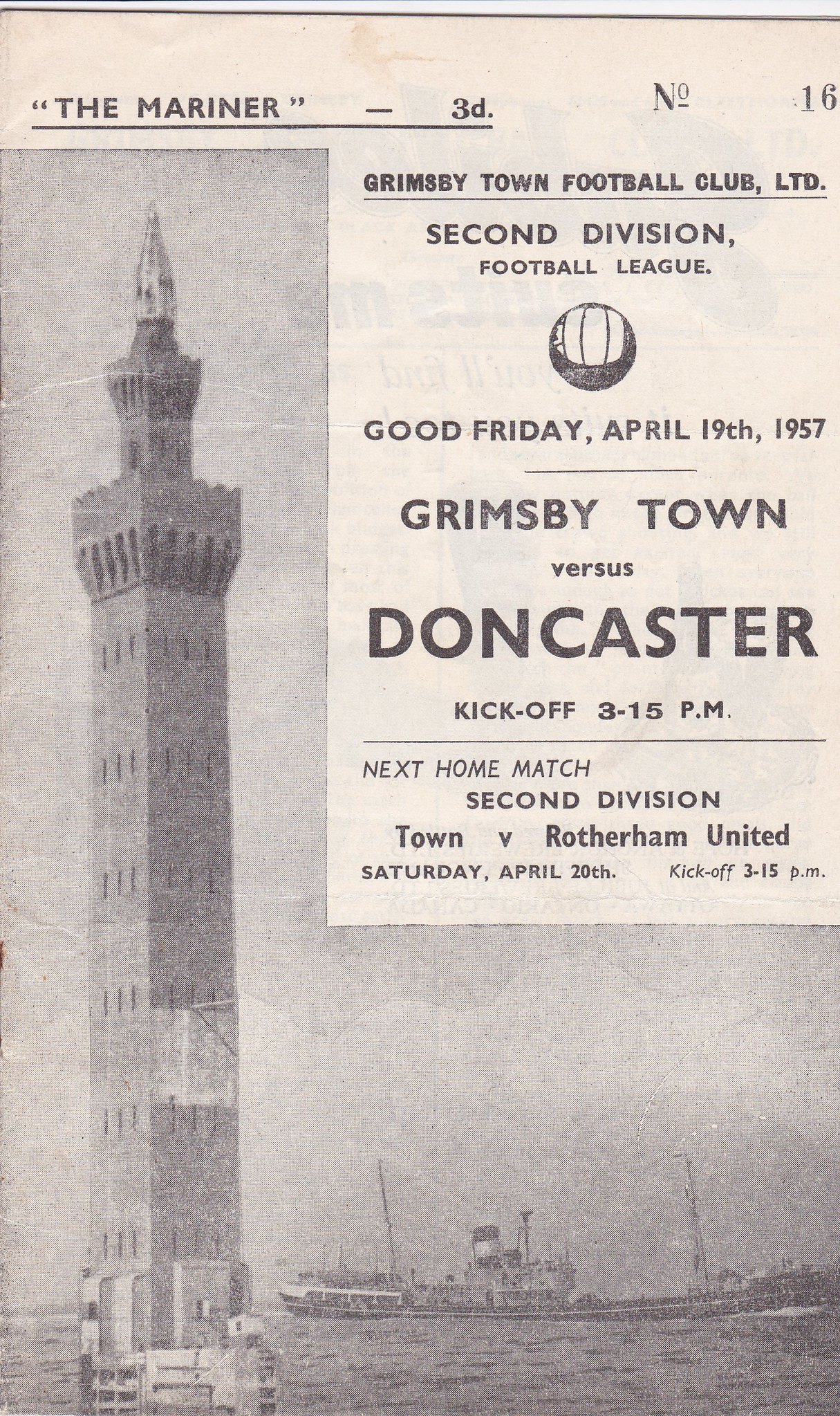This is a vertically oriented scan of an off-white, beige-tinted page from an old sports program, likely a pamphlet or magazine. The top section features the text "The Mariner," underlined and in black, followed by "3D," indicating the price in pre-decimalization British currency. The number "16" is positioned in the upper right corner, suggesting it is page or issue 16. Central to the page is a headline announcing "Grimsby Town vs. Doncaster," with the kickoff time set for 3.15 PM. A note below mentions the next home match, "Town vs. Rotherham United." The page is dated Good Friday, April 19, 1957, and belongs to the "Second Division Football League" under "Grimsby Town Football Club, LTD."

The bottom portion of the page is dominated by a black-and-white photograph of a tall, square stone tower emerging from the water, with a commercial ship, characterized by its central smokestack and low waterline, positioned to the right of the tower. This photograph, also black-and-white, adds a historic and nautical ambiance to the overall design.